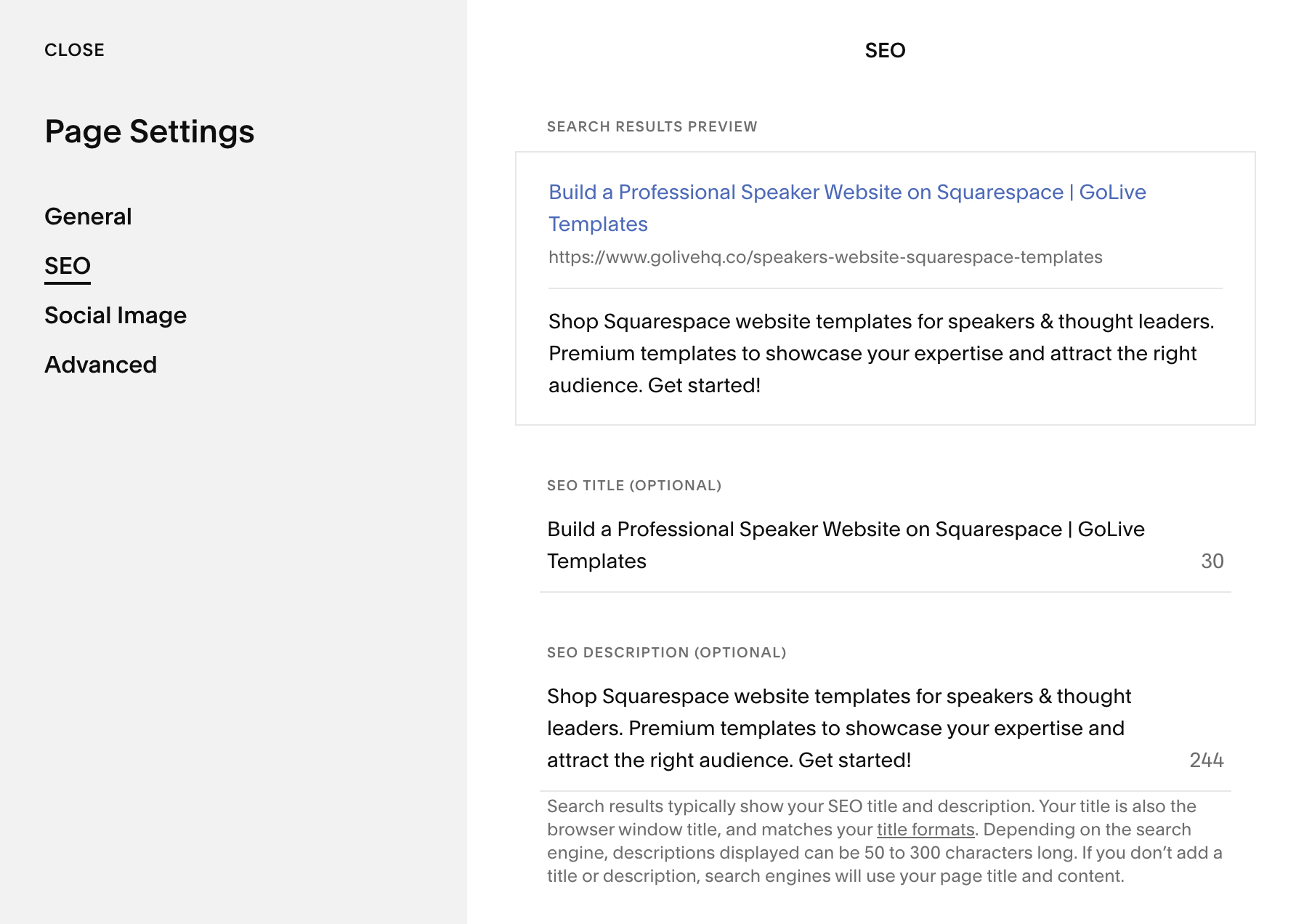The screenshot displays a section of a webpage interface, which appears to be part of a website builder or content management system.

On the left side of the interface, the sidebar features several menu options listed vertically. At the top, there is the command "Close.” About two inches below this, there is an option labeled "Page Settings." Further down, additional selections include "General," "SEO" (which is underlined), "Social Image," and "Advanced."

Transitioning to the right side, the main area is dominated by the "SEO" section header in uppercase letters. Directly below this, on the left, it reads "Search Results Preview." The preview displays how the site will appear in search engine results.

Highlighted in blue text, a sample title states, “Build a Professional Speaker Website on Squarespace.” Accompanying this title is a URL: "www.golivehq.co-speakerswebsitesquarespacetemplates." Beneath the URL, there is a brief description: "Shop Squarespace websites for speakers and thought leaders. Premium templates to showcase your expertise and attract the right audience. Get started."

In the next preview box, the title "SEO Optional" is shown, followed again by the text: “Build a Professional Speaker Website on Squarespace.” Finally, the last preview reiterates the description: "Shop Squarespace website templates for speakers and thought leaders. Premium templates to showcase your expertise and attract the right audience. Get started."

To the far right of this entire section, prominently displayed, is the number "244" followed by approximately four sentences in light gray text, which are partially obscured in this summary.